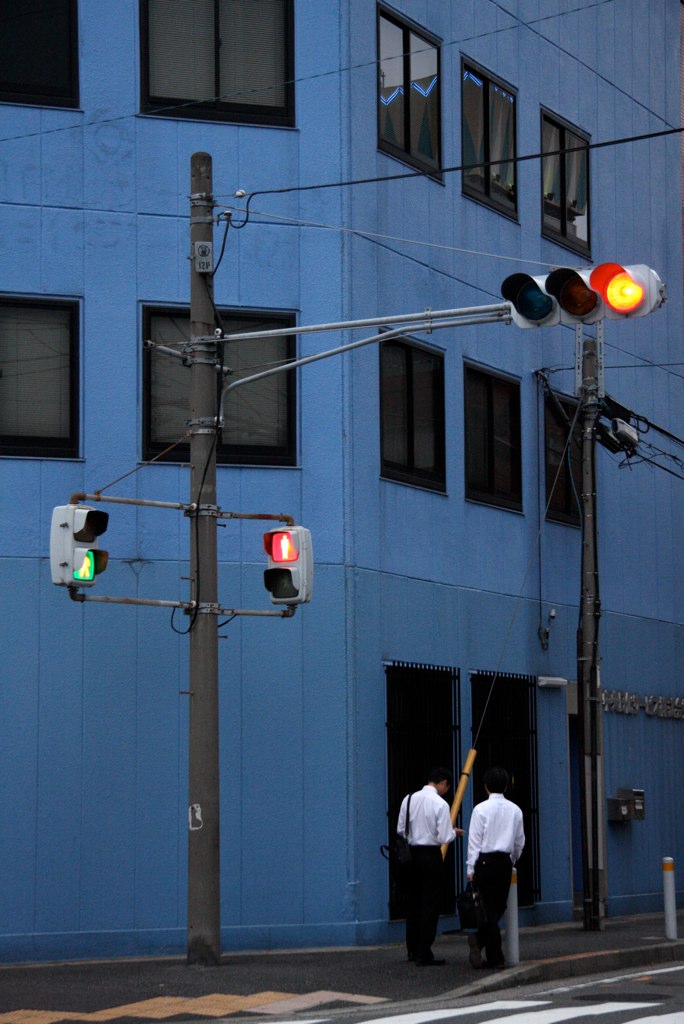The photograph, captured at dusk, depicts an urban street scene with a sidewalk in the foreground and part of a crosswalk visible at the bottom of the image. Two men dressed in white long-sleeve dress shirts and black pants stand just off the curb. The man on the left carries a bag slung over his right arm and left shoulder. Both gentlemen appear poised as if they might be engaged in conversation or waiting for something. A utility pole with walk-don't-walk indicators and a red stoplight are situated nearby. Behind the men, a large, multi-story building with dark gray and hint-of-blue, paneling and black-framed windows rises in the background. The building's windows are curtained, concealing the interior from view. The outdoor setting is completed with a network of power lines and cables crossing the scene overhead, contributing to the bustling urban environment.